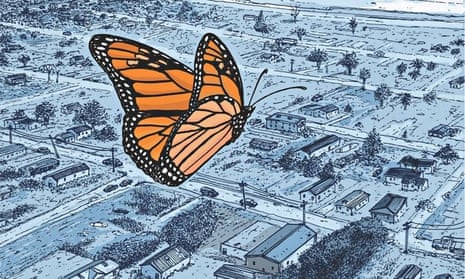This detailed illustration showcases a large, striking monarch butterfly, characterized by its vibrant orange wings, adorned with intricate black lines and white polka dots around the fringes. The butterfly, with its two slender antennas and delicate black body, is set against a painted rural landscape, seemingly flying at a considerable height. Dominating the composition, it occupies around 20% of the visual space, giving an impression of either a giant butterfly or a closer perspective compared to the backdrop.

Below, a serene, sparsely populated town unfolds, marked by a grid-like pattern of streets and avenues. The area is highlighted with small houses featuring gray rooftops, interspersed with trees and bushes, contributing to its rustic charm. The land is rendered in predominantly blue hues, suggesting a cold or wintry scene, possibly corroborated by the presence of white patches that might be snow-covered lawns. The town is not heavily populated, as seen by distinct open spaces and relatively few buildings. Adding to the quaint rural atmosphere, cars move along the streets which also feature telephone poles with wires, further enriching the painted scenery’s intricate details.